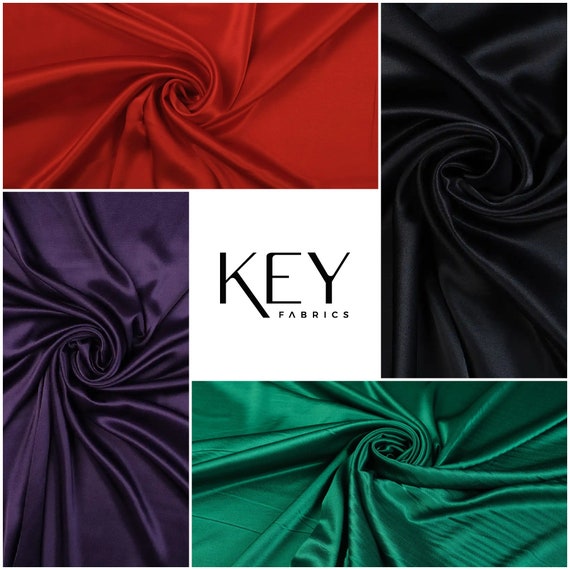This advertisement photo for Key Fabrics is designed in a square format with a clean, white background. At its center is a red square featuring the word "KEY" in bold, black capital letters, with "fabrics" under it in smaller black font. Surrounding this central square are four rectangles, each showcasing different colored satin or silk fabrics with a distinct swirling pattern that resembles a rose in the middle and lines of crumpled fabric extending outward.

- In the top left is a red satin fabric, twisted elegantly in the center.
- The top right displays a vertically oriented black satin fabric, also twisted centrally.
- The bottom right features a horizontal green satin fabric, similarly twisted in the middle.
- The bottom left shows a vertically aligned purple satin fabric, twisted in the center.

Each fabric piece adds a rich, luxurious texture, emphasizing the delicate and high-quality nature of the fabrics advertised by Key Fabrics.